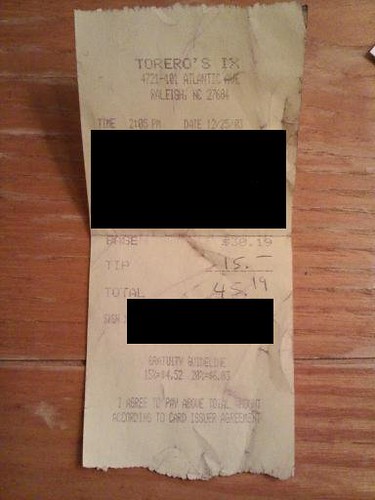This photograph captures an aged and wrinkled receipt from a restaurant called "Toreros," located on Atlantic Avenue in North Carolina. The receipt has evident signs of wear, including creases and what seems to be prior crumpling. Several portions of the document have been digitally obscured with large black rectangles, while a smaller black rectangle appears toward the bottom. The white receipt, featuring dark blue text, indicates that the customer left a generous $15 tip on a $30.19 order, totaling $45.19. The receipt rests on a wooden surface, likely a desk or table, further emphasizing the everyday nature of this captured moment.